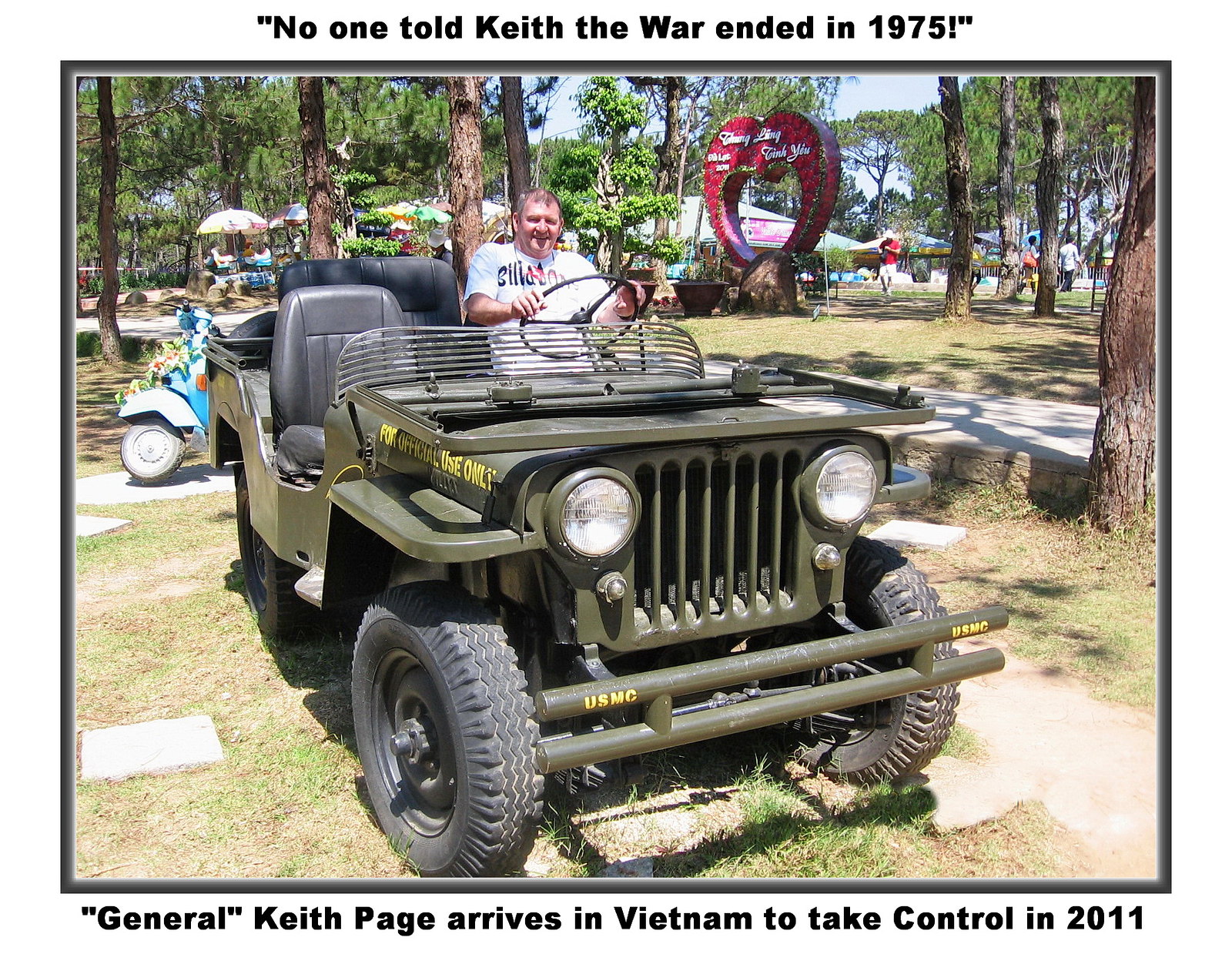In this photograph, an older white male, dressed in a white t-shirt with black writing, is sitting in the driver's seat of a vintage military vehicle, likely a Jeep, with an olive green exterior. The vehicle appears to be meticulously maintained, suggesting it might have been restored by the man himself. He is smiling cheerfully at the camera, holding one of the vehicle's thin wheels. The setting is an outdoor event, possibly taking place at fairgrounds or a park, noticeable by the large grassy area, scattered trees, and various tents, canopies, tables, chairs, and booths in the background. Among these, a prominent heart-shaped structure with white cursive writing stands out, likely serving as a decorative piece or a walking frame. The scene is bright and sunny, enhancing the nostalgic feel of the photo. Text overlay at the top humorously reads "No one told Keith the war ended in 1975," while the bottom caption states "General Keith Page arrives in Vietnam to take control in 2011," adding a playful and fictional narrative to the snapshot.